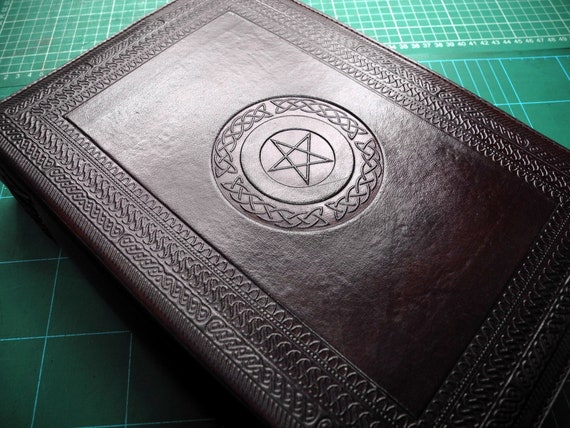The image depicts a dark brown, leather-bound book with a smooth, shiny cover that exudes an air of mystery and significance. The book's cover is adorned with intricate scrollwork engraved along its edges, which forms a beaded, braided-looking fringe. At the center of this ornate design lies a raised, embossed circle that houses a prominent star. The star, which has been described as both a Jewish star and a five-pointed star, is silvery and reflective, adding to the book's striking appearance. The book is void of any written inscriptions on its cover, contributing to the ambiguity of its contents—it could be a piece of religious scripture, perhaps a Torah, or something as enigmatic as a book of magic. The book rests on a green table with white lines, illuminated by overhead light, casting shadows that highlight its detailed craftsmanship.